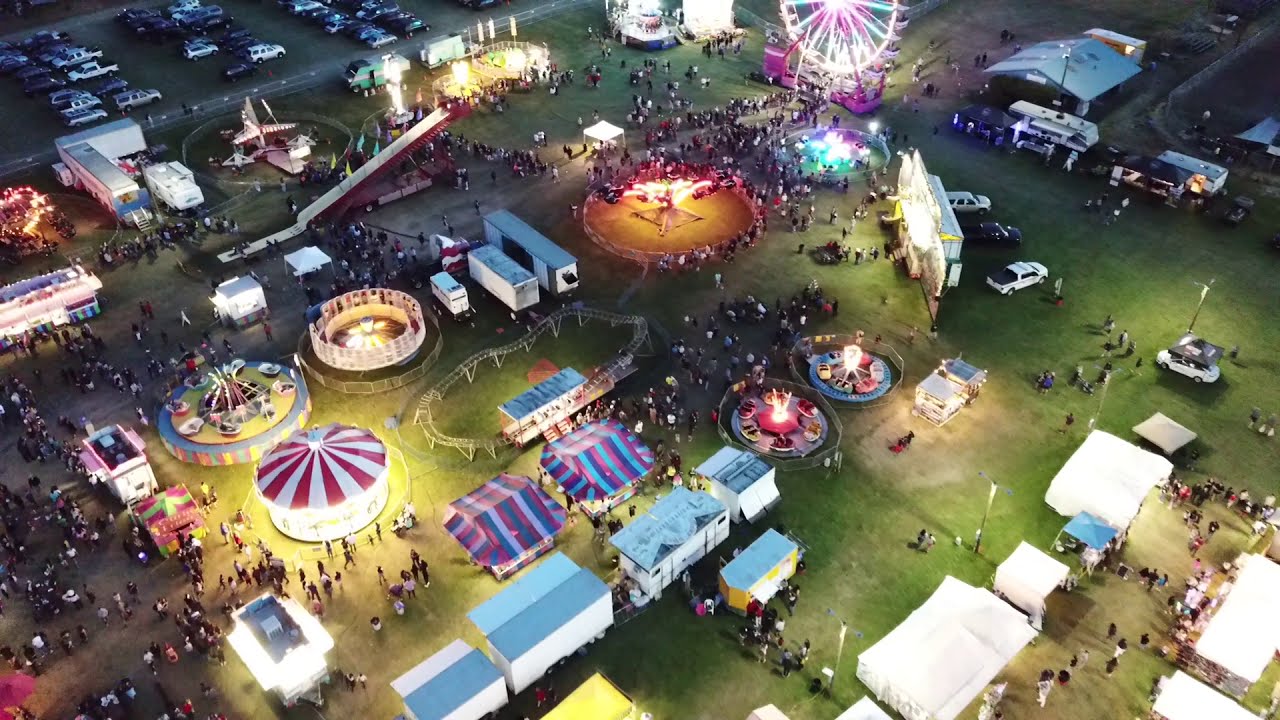This aerial image captures a vibrant fairground set against a dusk sky, transitioning into a summer evening. The left corner of the image features a bustling parking lot filled with a variety of vehicles, including white, silver, brown, and blue cars, while a nearby street provides access. The fairground itself sprawls out across grassy terrain, teeming with a large crowd of people navigating through the attractions. 

At the upper right center of the image stands a prominent Ferris wheel illuminating the scene with purple, blue, and white lights. Towards the lower left corner, a merry-go-round with a distinct red and white striped canopy catches the eye, surrounded by additional structures in red, blue, and dark blue hues. 

A roller coaster snakes through the middle of the carnival, its white tracks creating contrasting swirls against the darker ground, while a tilt-a-whirl and what appears to be a slip-slide ride add variety to the mix. Smaller rides and architectural structures, including tented buildings and trailers, are scattered around the edges, contributing to the fair's lively atmosphere. 

The whole scene is bathed in colorful lights, with rooftops showcasing patterns in red, white, purple, and blue, and ride cars in vibrant shades of yellow, red, white, and silver. The extensive illumination and bustling activity make it clear that this is a well-attended, lively carnival event.